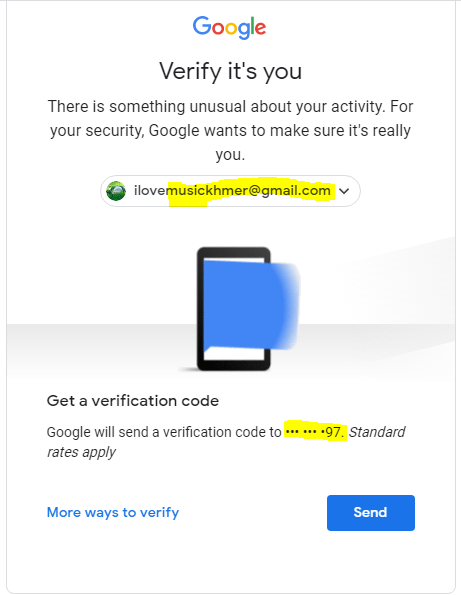This image depicts a Google verification window. At the center top of the screen, the iconic colored Google logo is prominently displayed. The screen itself is predominantly white, bordered by a fine gray line, with the lower half featuring a very light gray color.

Just below the Google logo, the words "Verify it's you" appear in a larger font. Beneath this, smaller text reads, "There is something unusual about your activity. For your security, Google wants to make sure it's really you." Under this, there is a pull-down list containing an email address, "ilovemusichmer@gmail.com," with the portion "musichmer@gmail.com" highlighted in yellow to draw attention.

Further down, there is an image of a smartphone with a blue streak across its center. The gray panel that I mentioned earlier holds additional informational content. It bears a heading that reads "Get a Verification Code." The text below explains that Google will send a verification code to a partially obscured phone number ending in "97," with a note that standard rates apply. To the left, a hyperlink titled "More ways to verify" is available for users seeking alternative methods to receive the code. On the right-hand side, a clearly marked "Send" button is visible, which, when clicked, will dispatch the verification code to the indicated phone number.